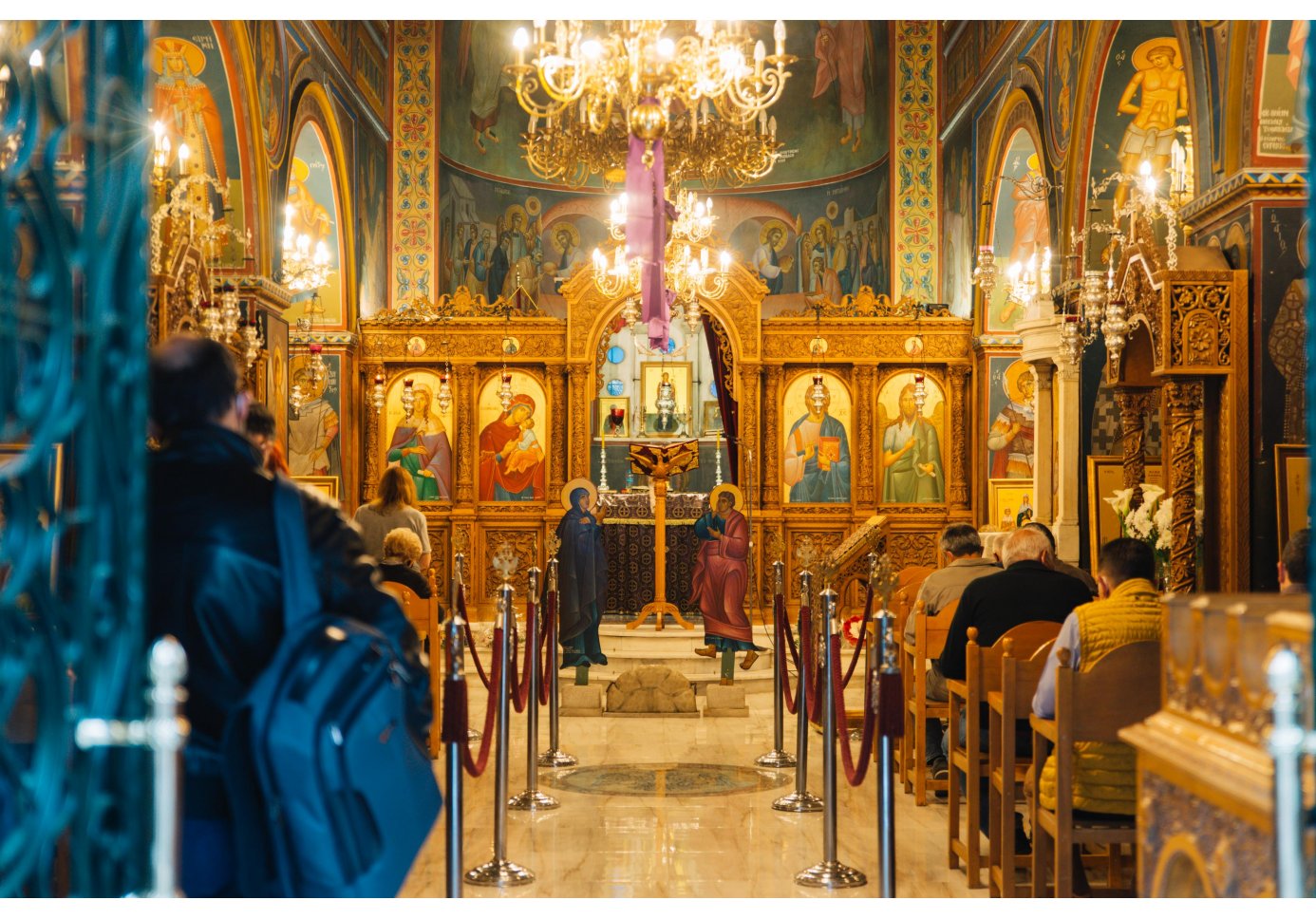The photograph captures the opulent interior of a grand cathedral, likely visited by tourists. At the forefront, a central aisle is framed by silver poles connected by red velvet ropes, guiding the flow of visitors and blocking off certain sections. On the right side, wooden chairs or pews are filled with worshippers, and a lattice door reveals a man in a black leather jacket with a blue backpack. The cathedral's interior is adorned with intricate gold decorations, exuding an aura of elegance. The walls are embellished with Renaissance-style paintings of biblical figures, including Jesus, Mary, and the baby, set within curved arches. Dominating the ceiling is a magnificent gold chandelier, bathing the space in bright light. The ceiling itself is a canvas of detailed paintings, further enhancing the sacred atmosphere. The meticulous woodwork, archways, and overall grandeur underscore the cathedral's sanctity and historical significance.